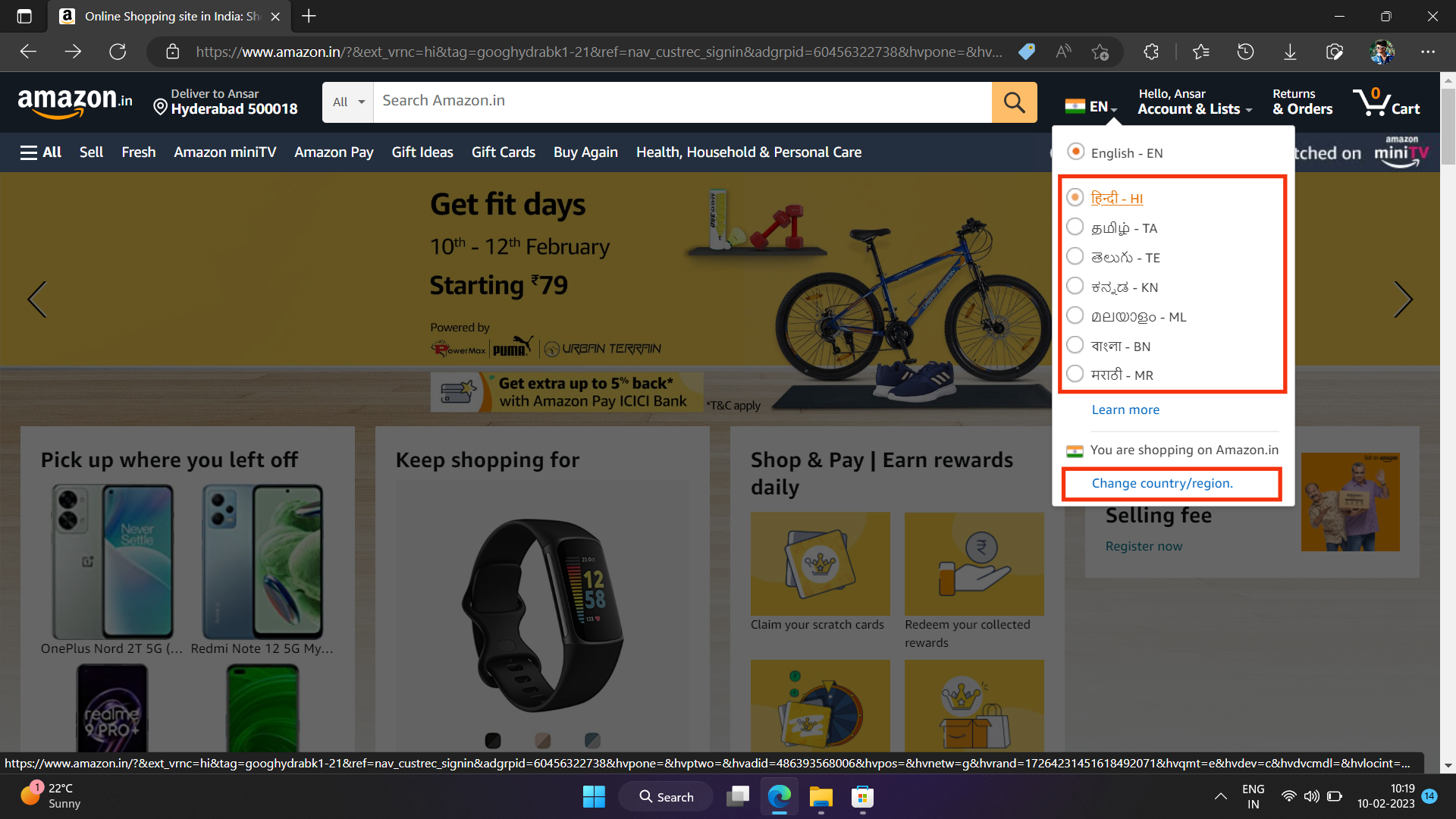**Detailed Caption:**

This screen capture appears to be from the Amazon.in website accessed via Mozilla Firefox. The browser's tab, which is gray and selected, indicates an online shopping site in India. On the left-hand side, the Amazon logo is displayed within a white square, featuring a black lowercase 'a' with a gold swoosh underneath. 

Adjacent to the logo, there are white forward and backward navigation arrows and a refresh icon, all set against a dark gray bezel. The URL bar, also in a dark gray oval, features a white padlock icon followed by the darker gray text "https://" transitioning to white text "amazon.in". 

Further, the URL bar extends into a gray string of text, indicating the long website address. On the extreme right side of the URL bar, there are several icons: a gear, a star with lines (likely for bookmarking), a clock (possibly for history), a down arrow, and a camcorder icon. 

Below the address bar, the webpage header displays "Amazon.in" next to a delivery location set to Hyderabad (PIN: 5000018). A series of tabs including "Sell," "Fresh," "Amazon miniTV," "Amazon Pay," "Gift Ideas," "Gift Cards," "Buy Again," and "Health, Household and Personal Care" are present, all written in white text.

An Indian flag is shown to the right, comprising horizontal bands of orange, white, and green with a central symbol, possibly the Ashoka Chakra, too small to discern clearly. Next to it is the "English - EN" language setting. A dropdown reveals additional selectable Indian languages denoted by their respective abbreviations in blue text: "HI", "TA", "TE", "KN", "ML", "BN", "MR".

Highlighted clickable text reads "Learn More". Adjacent to this text, "You are shopping on Amazon.in" and a selected option with a dropdown contain a red rectangle, showing the option to "Change country/region" in hyperlink-style blue text.

On the far right part of the dark blue bezel, there are welcoming texts: "Hello, NSAR" indicating the user, alongside links for "Returns & Orders" and a shopping cart icon displaying "0" items in bright orange, denoting an empty cart.